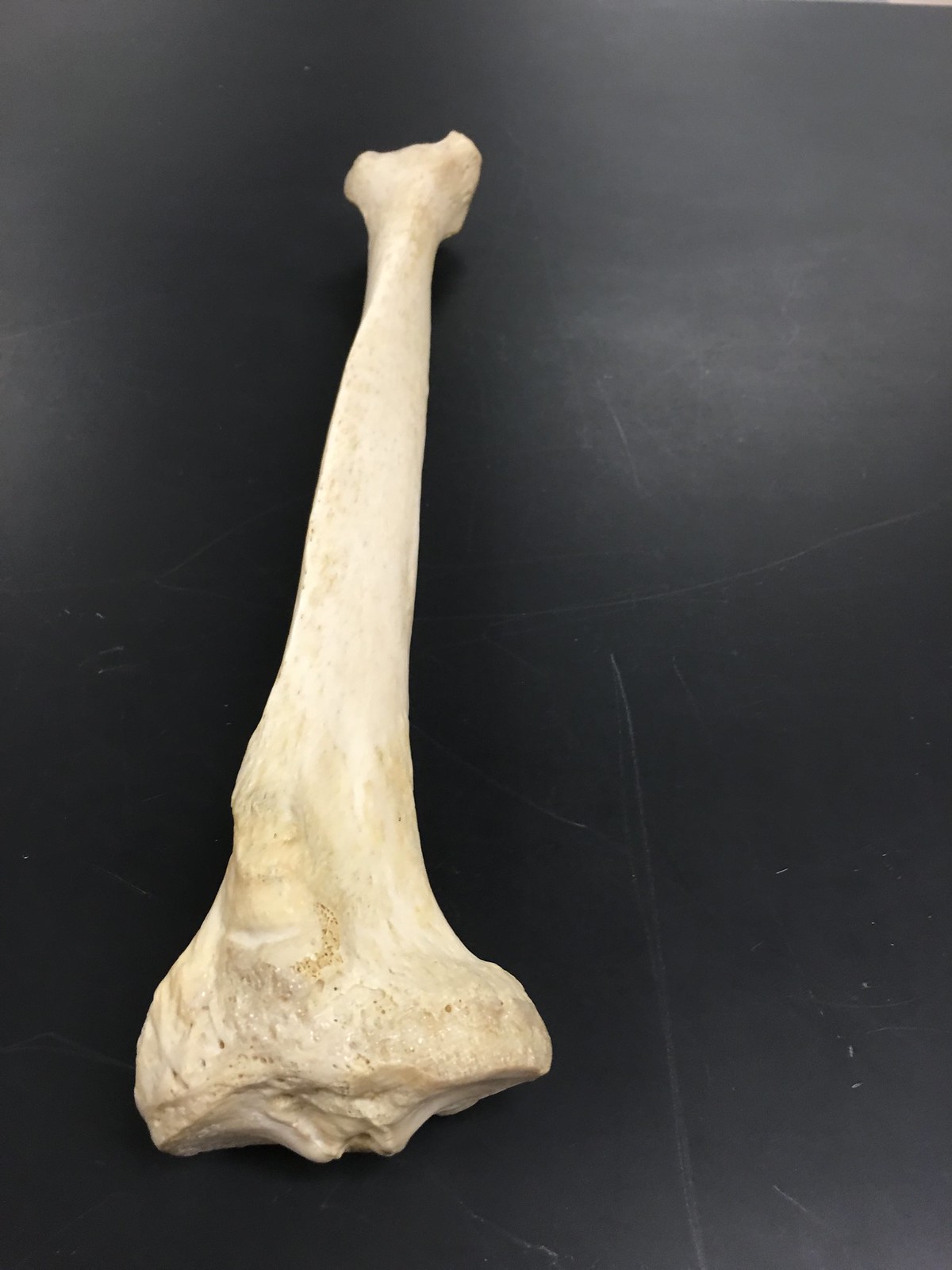This image features a long, slightly cream-colored bone with a tan or whitish-brown hue, lying on a solid black background. The bone appears slightly off-center in the frame, surrounded by a border of approximately two inches at the top and bottom. The bone is notable for its irregular shape, starting relatively narrow at the top, then gradually widening and flaring out towards the bottom, where it ends in a rough and wider section. This uneven texture at the wider end contrasts with the smoother but still slightly speckled and shiny surface elsewhere, highlighted by artificial lighting. The bone could be from a mammal, potentially including a human, and might be a leg or arm bone based on its shape and structure.